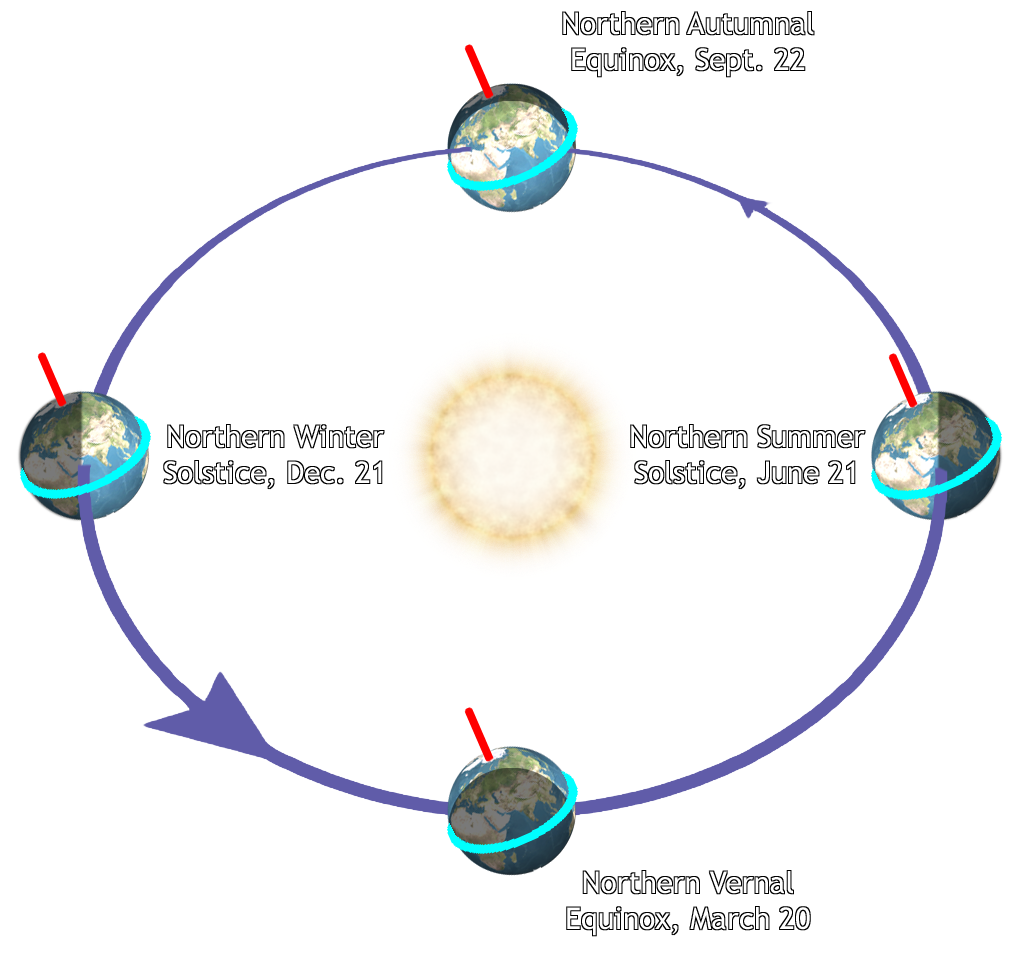This detailed color illustration, in landscape orientation, features the rotation of the Earth around the Sun at various points throughout the year. The background is white. At the center of the image is a white-yellow Sun with a diffused gold aura. Surrounding the Sun is a dark blue elliptical circle with arrows pointing counterclockwise, connecting four images of Earth positioned at different points along the ellipse.

1. At the top, labeled in white text outlined in black, is the "Northern Autumnal Equinox, September 22nd." This Earth image shows a blue equatorial ring and a red line indicating the North Pole, angled to the top left with a crescent shadow on the upper portion.

2. To the left, similarly labeled, is the "Northern Winter Solstice, December 21st." This version of Earth has a black shadow on the left side.

3. At the bottom, labeled "Northern Vernal Equinox, March 20th," the Earth shows a shadowed hemisphere facing the viewer, with only the part nearest the Sun illuminated.

4. To the right, labeled "Northern Summer Solstice, June 21st," the Earth is half-lit on the inside part facing the Sun, while the far-right part is in darkness.

Each Earth image is tilted on its axis, indicated by the red line projecting from the North Pole, showing how the Earth's tilt and resulting shadows vary throughout the year. This richly colored, multi-element educational piece accurately illustrates the Earth's position relative to the Sun and the shadow's movement during the equinoxes and solstices, emphasizing the cyclical nature of our planet's solar orbit.